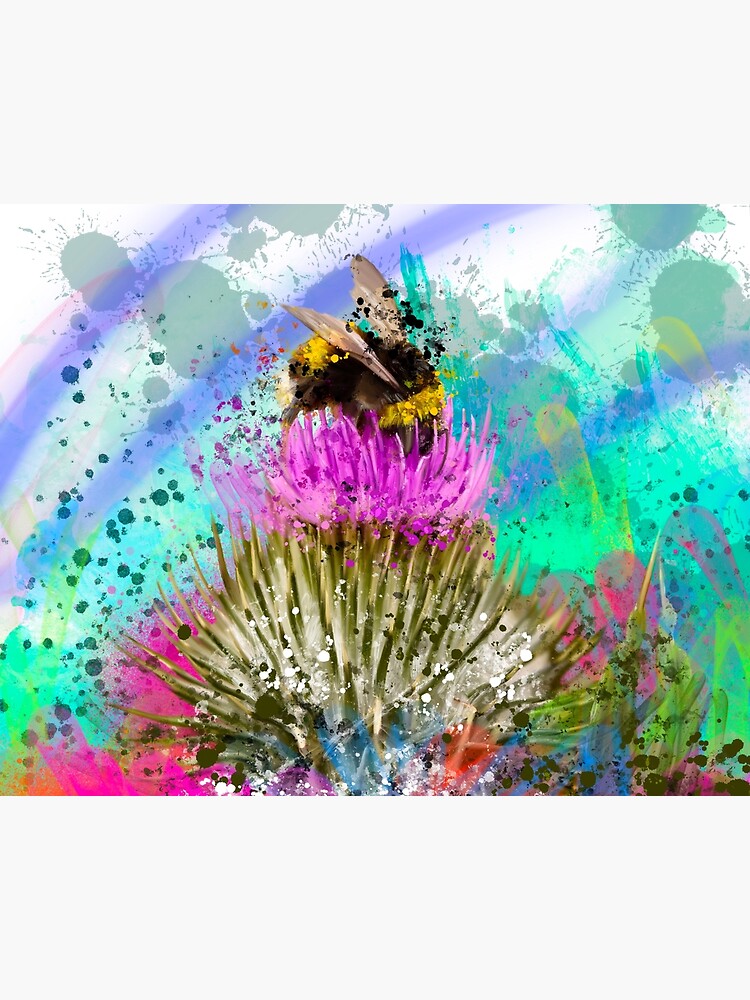This abstract watercolor painting features a vibrant and dynamic composition. The background is adorned with several blue curved lines and is richly punctuated by splashes of various colors, including green, light green, pink, yellow, dark pink, and multiple shades of blue. The splashes form circular patches that complement the central figure of a flower. The flower has slender, long green and white leaves at the base, supporting a large, prominently positioned pink bloom. Atop the pink flower rests a bee with distinctive yellow and black stripes on its body and two brown wings. The background is a technicolor array of specks in green, red, pink, and white, lending a uniquely splattered yet harmonious aesthetic to the image.